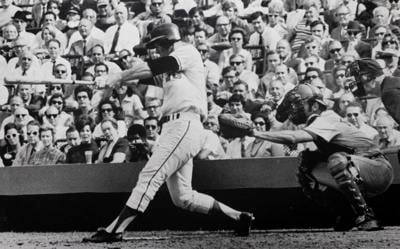This black and white photograph captures a dynamic moment from a baseball game, presented in a wide, slightly vertical rectangular format. At the center of the image, a batter, donned in a white uniform with dark shoes and a helmet, is captured in mid-swing. His hands clasp the bat, which arcs around his body and extends in front of him, indicating a powerful follow-through. Behind the batter, the catcher crouches with knee pads, a face mask, and a hard hat, his gloved hand outstretched, poised to catch the ball if the batter misses. The field extends below, and a solid rectangular wall frames the background, where a diverse crowd sits shoulder to shoulder in the stands. Men and women of various ages, many wearing sunglasses, are attentively watching the game in the daylight. The overall scene, devoid of any text or words, vividly conveys the intensity and communal atmosphere of a daytime baseball game.